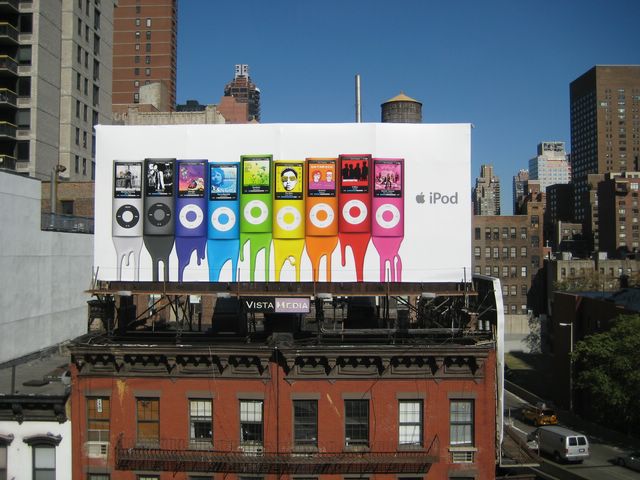In this vibrant cityscape, an eye-catching billboard proudly advertises the iPod atop a charming red brick building with dark grey trim. The sleek white banner features nine iPods, neatly aligned side-by-side, showcasing a spectrum of colors: light grey, dark grey, dark purple, light blue, green, yellow, orange, red, and pink. Each iPod displays a unique image on its screen and is equipped with the iconic circular controls. To the right of the colorful array, the billboard prominently displays the Apple logo next to the word "iPod." Below this central image, a sign reads "Vista Media," adding another layer to the urban scene. Surrounding the building, there are taller high-rises in varying shades of grey and dark brown, framing the snapshot of the blue sky above. On the street below, a grey van drives past a tree and a streetlight, integrating the dynamic elements of city life into the advertisement's setting. The dripping color effect beneath each iPod accentuates their hues, making the advertisement both vivid and memorable.